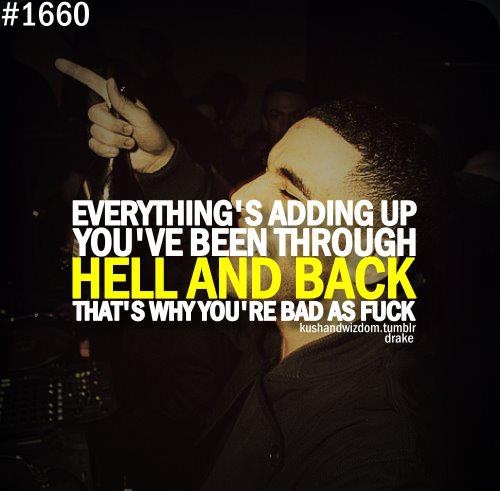This is a vibrant and striking color image commonly circulated as a meme or inspirational graphic. Dominated by a predominantly black background, the focal point of the image is a young adult male, identified as Drake, with his eyes gently closed, evoking a sense of calm or introspection. Drake is dressed entirely in black, which harmonizes seamlessly with the dark backdrop and adds to the intensity of the image. 

Adorning the top left corner of the image is the text "#1660," seemingly a reference number or tag. Enhancing the emotional tone, overlaid text spans across the image with a powerful message: "Everything's adding up. You've been through hell and back. That's why you're bad as fuck." This statement speaks to resilience and strength, amplifying the inspirational impact of the graphic. 

The source of the image is indicated at the bottom, where "K-U-S-H-A-N-D-W-I-Z-D-O-M.tumblr" is credited, denoting it as a Tumblr post. Additionally, the name "Drake" is mentioned underneath, affirming the subject's identity. This carefully crafted post combines visual and textual elements to deliver a poignant, motivational message.